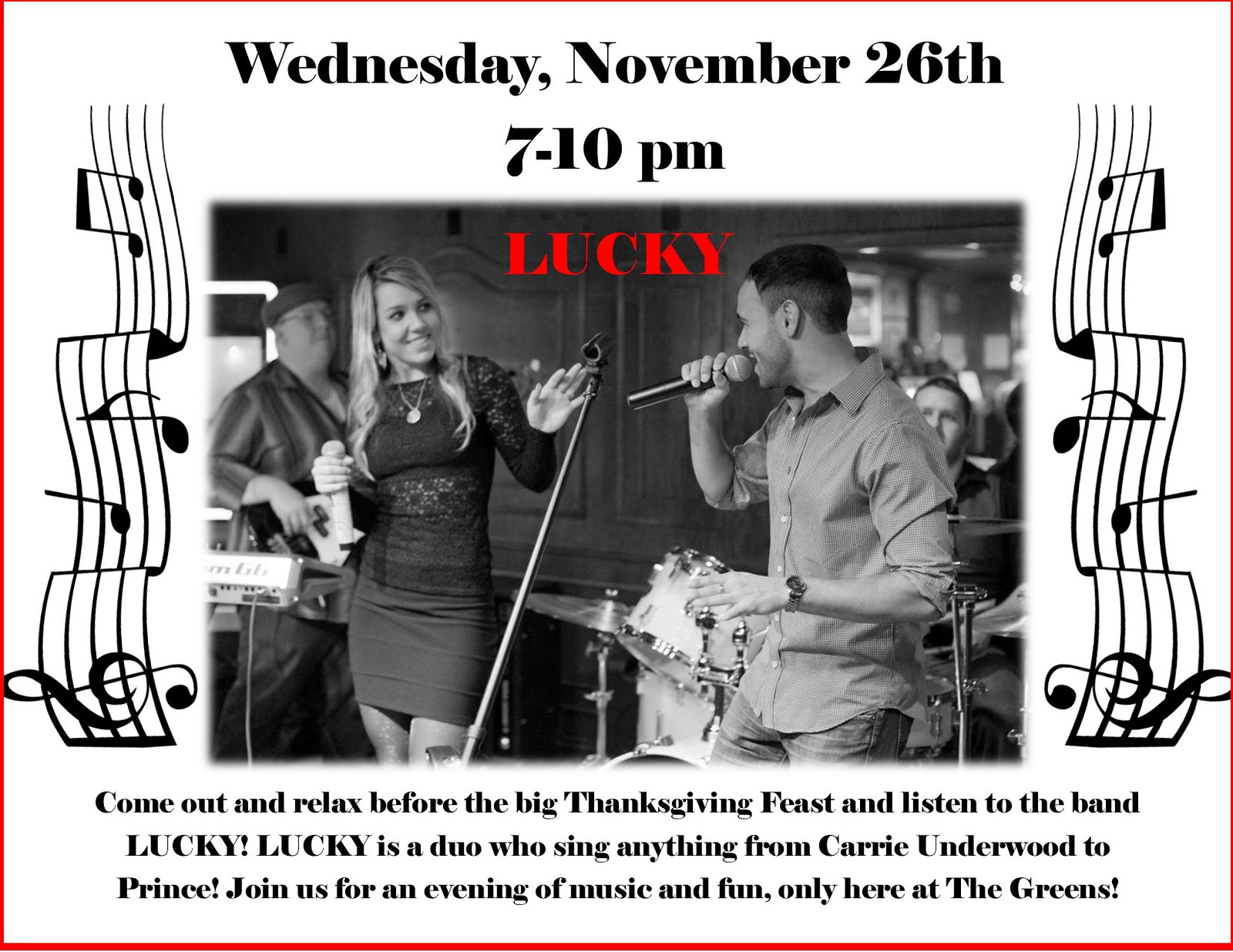This local advertisement features a square image bordered by a thin pinstripe red outline against a white background. Prominently displayed at the top in bold black print is the event date and time: "Wednesday, November 26th, 7-10 p.m." Below this is the focal point of the ad: a black-and-white photo capturing a live music performance.

On the right side of the photo stands a man with short black hair and a closely cut beard, wearing a long-sleeve gray button-up shirt rolled up to his elbows and blue jeans. He holds a microphone in his right hand, which is raised, as he sings and faces towards the left. Behind him, a seated person is visible, playing a white drum set.

To the left in the same photo, a long-haired blonde woman, dressed in an elegant, lacy black dress and a necklace with an emblem, stands holding a microphone down by her waist with her right hand. Her left hand is lifted with its palm facing out. Behind her, a man with glasses, a gray hat, and a long-sleeve shirt plays a bass guitar.

Centrally placed above the photo in bold red print is the word "Lucky." Flanking both sides of the image are vertical rows of music notes, adding a musical theme to the ad. 

At the bottom, the ad invites viewers to a special pre-Thanksgiving event with this enticing message: "Come out and relax before the big Thanksgiving feast and listen to the band Lucky. Lucky is a duo who sing anything from Carrie Underwood to Prince. Join us for an evening of music and fun, only here at The Greens."